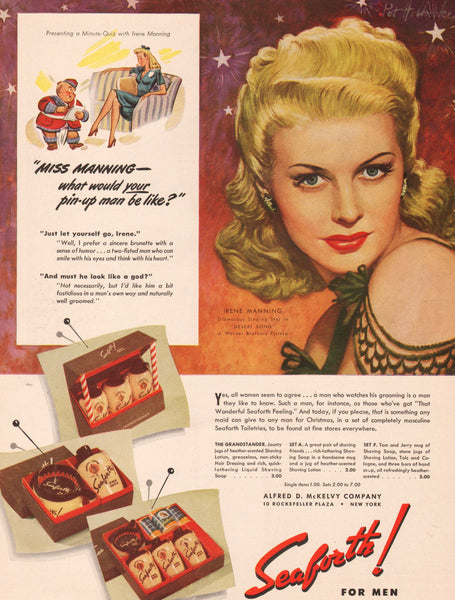This appears to be a vintage magazine advertisement from the late 1930s to early 1950s. The ad is rectangular and features two main sections. The top three-quarters of the ad has a reddish background that gradates to orange, adorned with light red or pink stars. In the top left corner, a small round man in a red jacket and matching hat stands beside a woman sitting on a couch, dressed in a blue uniform, possibly a stewardess. A headline next to their image reads, "Miss Manning, what would your pin-up man be like?" 

To the right, the prominent face of a blonde-haired woman with red lips and blue eyes looks towards the camera over her shoulder. She is wearing some sort of designer, possibly off-shoulder, attire. This woman is likely Irene Manning, as her name appears in the ad. Below her image, the background transitions to a light pinkish tan, where smaller images of jars or cans, possibly of toiletries like cologne, are pinned up. Some additional text indicates these products are part of the C4 line, meant specifically for men.

At the bottom right corner, the tagline "C4! For Men" is prominently displayed, and nearby text suggests the products are branded as masculine grooming essentials ideal for a Christmas gift. The ad concludes with a mention of the brand and company name: "Alfred D. McAvee Company, 10 Propeller Plaza, New York," all in red-colored fonts.